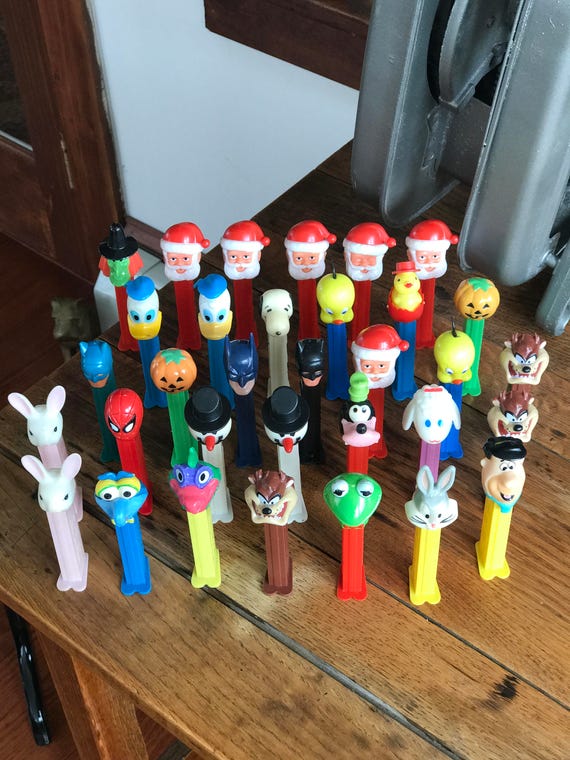This image showcases a diverse collection of 33 Pez dispensers arranged in five rows on a light-colored wooden table. In the back row, there are five Santa Claus dispensers depicted with white beards and red hats, accompanied by a green-faced witch with red hair and a black hat on the left side. In the second row, there's a variety of characters: two Donald Duck dispensers, Snoopy, Tweety Bird, a rubber ducky, and a jack-o-lantern. The third row continues the theme with Batman, another Tweety Bird, a second jack-o-lantern, Santa Claus, and Tasmanian Devil dispensers. Moving forward, the fourth row includes a Bunny, Spider-Man, two snowmen, Goofy, Lamb Chop, and another Tasmanian Devil. Finally, the front row features Fred Flintstone, an alligator, yet another Tasmanian Devil, a figure resembling Gonzo, Kermit the Frog, a second Bunny, and Bugs Bunny Pez dispensers. Each character is clearly detailed in this impressive collection, sitting neatly on the wooden table.